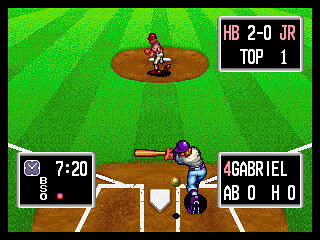The image depicts a vintage-style baseball video game, possibly designed for a smaller screen device. The game showcases an infield with green, vertically striped rectangles mimicking a meticulously mowed baseball field. At the center, a reddish-colored pitcher's mound features a pitcher wearing a red helmet, red cleats, white pants, and a pink shirt. The batter, positioned at the home plate on a similarly reddish mound, is captured mid-swing, wearing a purple helmet, blue jeans, white shirt, and purple cleats. The ball hovers just behind the batter, having narrowly missed the swing, passing over the home plate and the batter's boxes.

In the upper right corner of the screen, a black scoreboard displays "HB2-0JR, Top 1." The bottom left features a clock reading "7:20" and possibly indicating balls, strikes, and outs with "BS0" followed by a red dot. The bottom right corner reveals the batter's stats: "4 Gabriel, AB0H0," denoting the batter's number and performance metrics in the game. The entire scene is rendered in a low-resolution, classic video game style, evoking nostalgia for early gaming visuals while providing a detailed snapshot of the in-game baseball action.